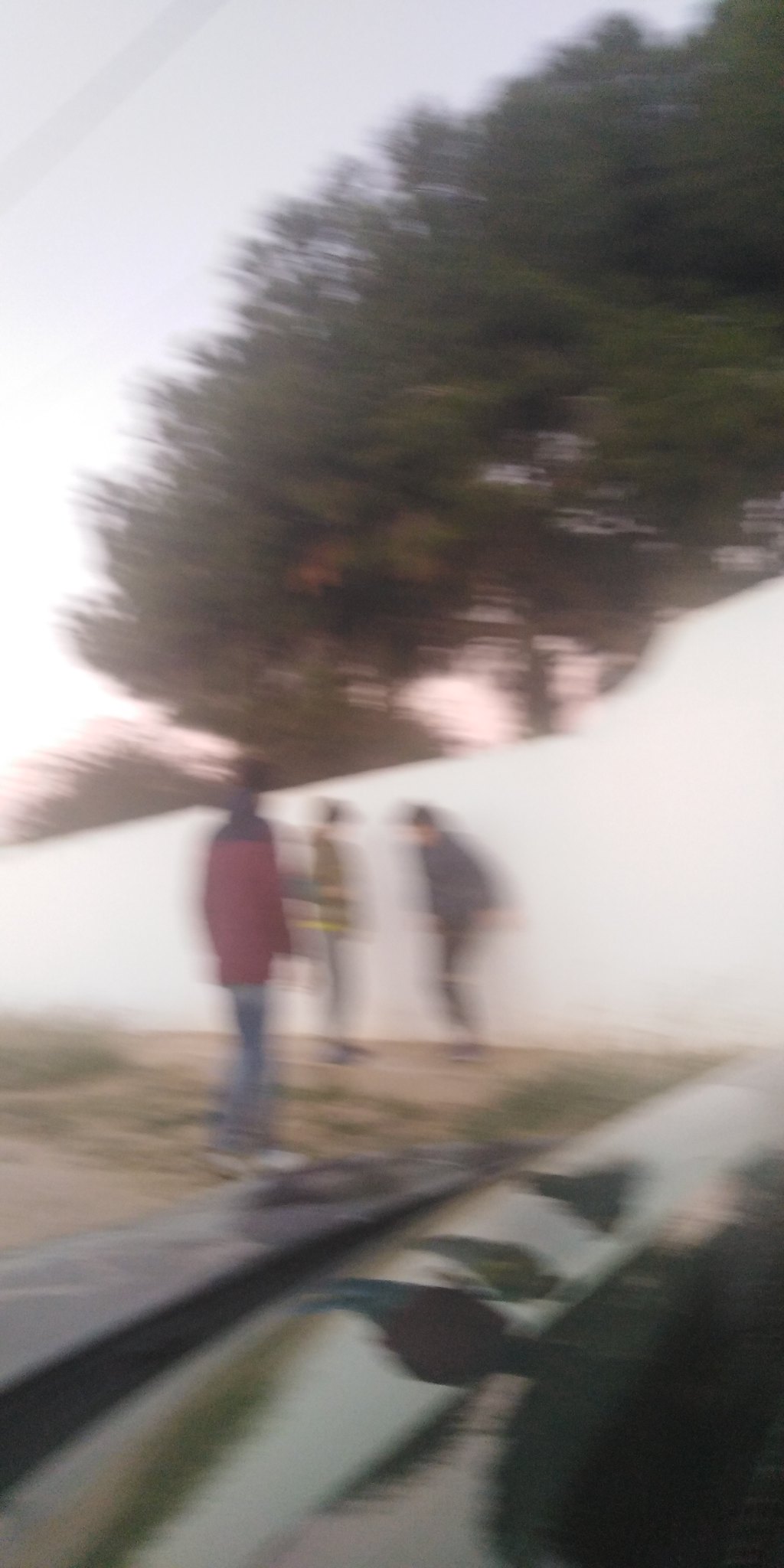This is a blurry, overexposed, vertical color photo taken outdoors, depicting three people. Two of the individuals are standing against a white wall, possibly a brick wall, with green trees and a pale sky, tinged with pink, visible above. One person in blue jeans and a red jacket with a black yoke across the shoulders has their back turned to the camera, wearing white tennis shoes and standing closer to the camera. The other two, positioned further back in front of the wall, are facing each other. One wears light-colored pants and a yellowish jacket, and the other sports a blue jacket and darker jeans. The ground appears to be dirt or sand, with some green patches, and there's an unclear reflective surface in the foreground, perhaps a car hood, showing faint reflections of the three figures. The image is of poor quality, making fine details indistinguishable.